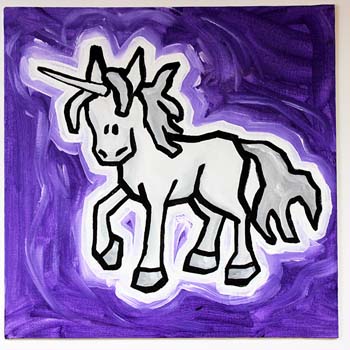The image is a detailed square painting featuring a small, white unicorn with delicate, black marker outlines. The unicorn is depicted in a side profile facing to the left, with two small dots for eyes and two dash lines for the nose. Its horn, forelock, and ears are all white, matching the main body. The mane, tail, and hooves are shaded in a light gray, adding subtle contrast to the unicorn’s figure. Surrounding the unicorn is a distinct white outline, which is further framed by a lavender hue. This fades seamlessly into a purply, dark purple background that displays visible brush strokes, evoking a sense of layered paint applied with expressive, sliding motions. The contrast between the white unicorn and the rich purple tones creates a striking visual effect, highlighting the intricate details of the mystical creature against the textured backdrop.